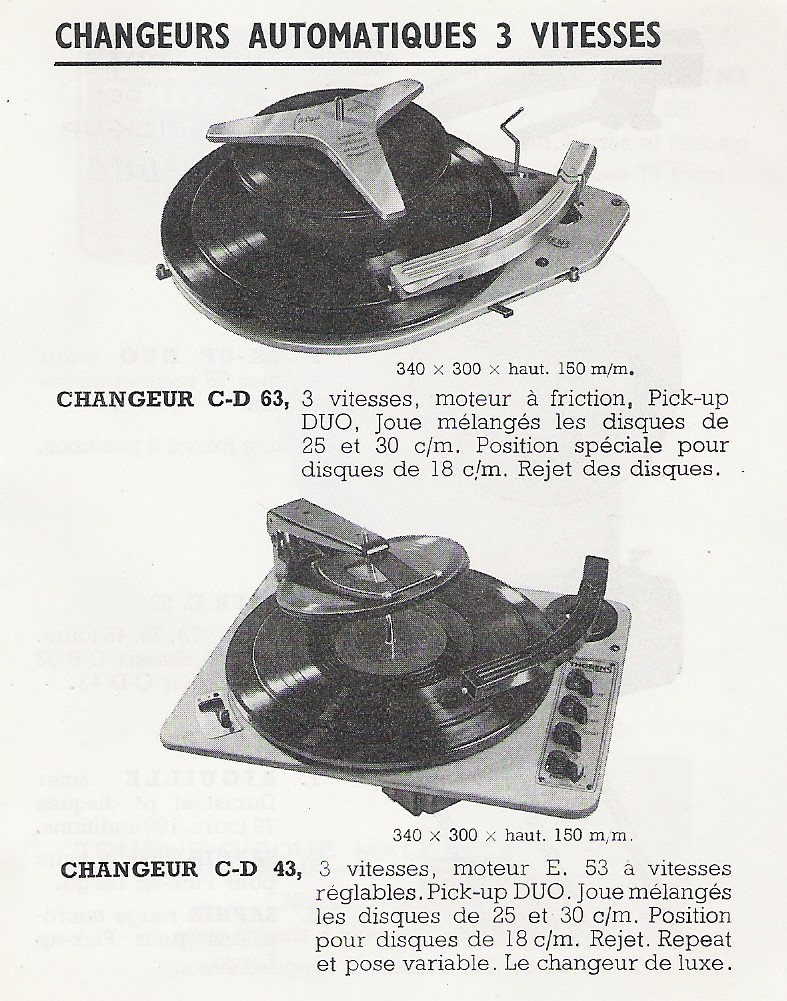The image is an old-time advertisement, presented on a white background, likely originating from a magazine or manual, as it seems highly detailed and informative. The text, entirely in French, provides information on different models of record players, referred to as "Changeurs Automatiques 3 Vitesse." At the top, bold and underlined text catches the viewer's eye, indicating the main focus of the advertisement.

Below this headline, there is a black-and-white image of a vintage turntable mechanism with a metallic arm positioned over a black vinyl LP. This turntable setup includes additional 45s held by an arm above the main record. Accompanying this image is a block of descriptive text in French, detailing the model and its specifications, including dimensions.

Further down the page, another image showcases a more modern turntable system, distinguishable by its numerous dials and advanced features, yet still adhering to a black and grey color scheme. This image is also complemented by a descriptive paragraph and model information, continuing the advertisement's pattern. The overall design and layout suggest a sophisticated marketing effort to highlight the evolution and features of these automatic record changers.